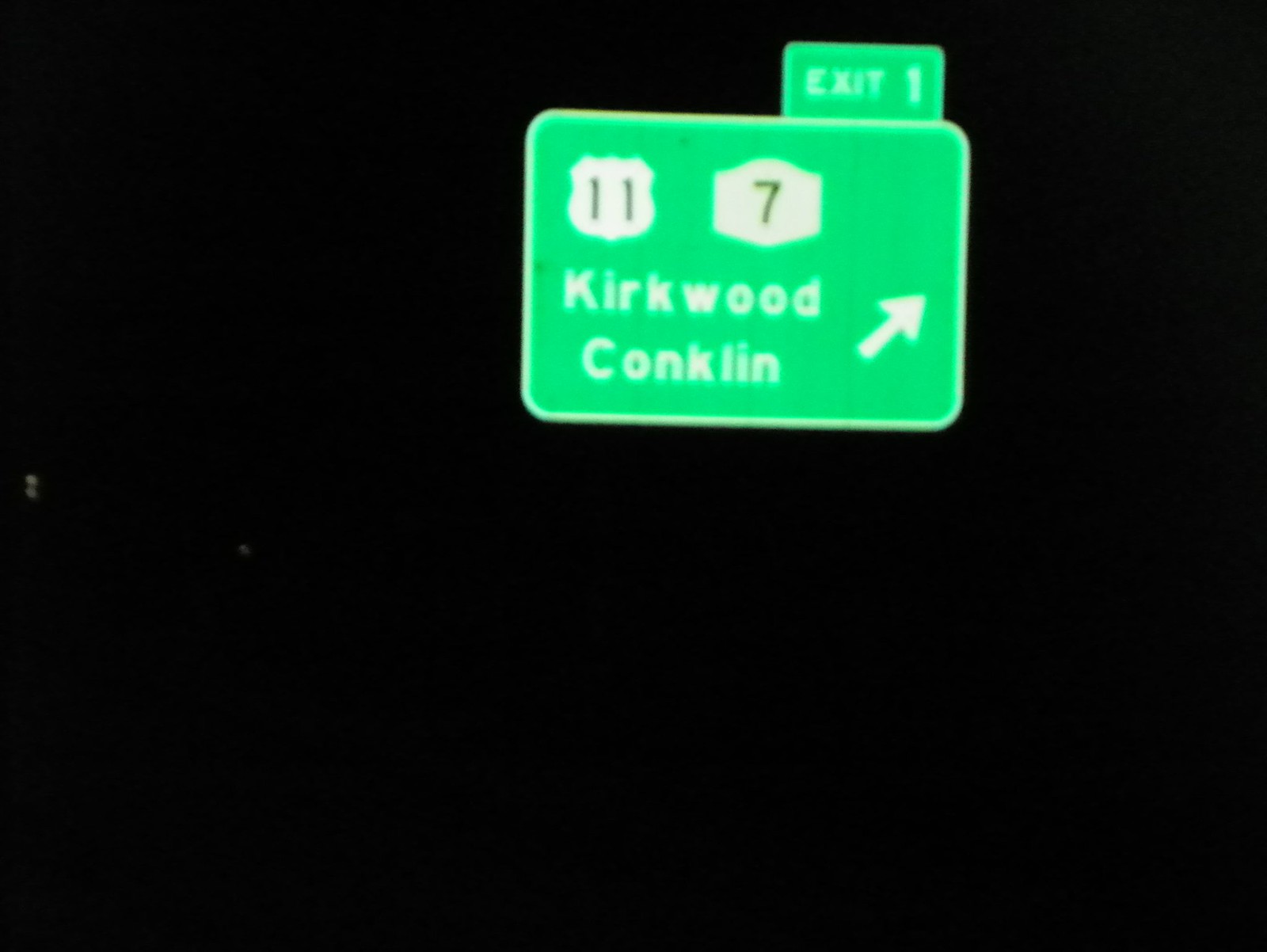The photograph captures a nighttime scene, predominantly shrouded in darkness. Toward the middle left of the image, three small white dots are visible, likely the headlights of oncoming cars. Above these lights, a green road sign stands out against the black background. This rectangular sign, with rounded edges, features key details in various shapes and colors. 

On the sign, a white crest-like emblem denotes an interstate, bearing the number 11 in black. Adjacent to it is another similar shape with the number 7 also in black. Below these emblems, the words "Kirkwood Conklin" are written in white, with an upward-pointing arrow indicating the direction. This arrow, angled slightly to the right, guides travelers rather than pointing directly upwards. Topping the sign is a small white square displaying "Exit 1" in clear, bold text. The green of the road sign provides a stark yet informative contrast to the deep black of the night.